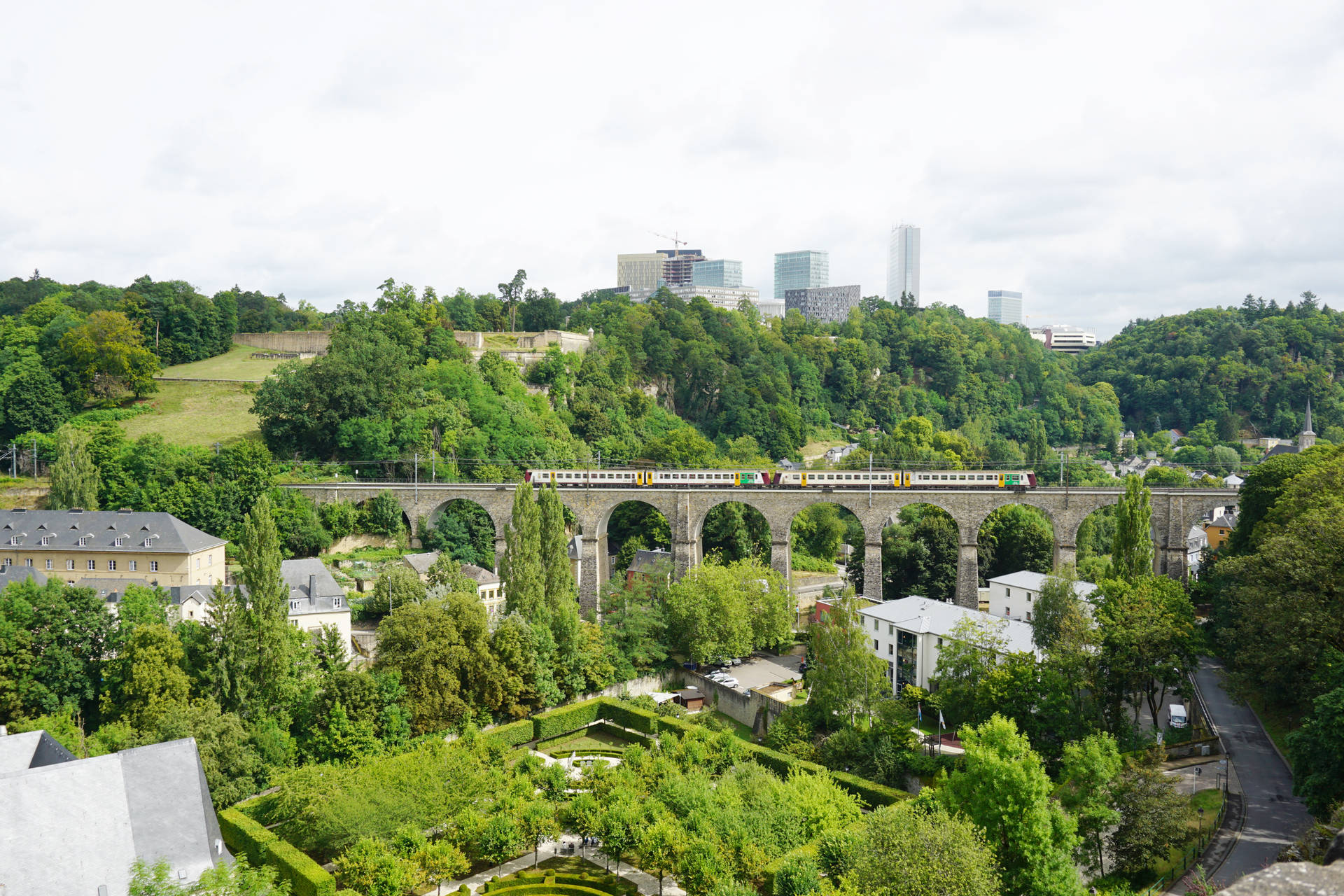This photograph captures a scenic view of a train journeying across what appears to be a Roman aqueduct, supported by large, circular pillars. The aqueduct spans over a lush valley teeming with verdant greenery, indicative of spring or summer. Amidst the foliage, a mix of buildings emerges, likely a combination of hotels, businesses, and city structures, adding to the urban charm. The train itself, comprising four sizable passenger cars, stands as the focal point, gracefully traversing the impressive stone structure. In the far distance, a cityscape unfolds with a striking skyline featuring two tall buildings and one dominating, slender skyscraper peeking through the trees. Above, a clouded yet bright sky, with white clouds and hints of grey on the right, blankets the scene in daylight. To the left, a prominent large building takes center stage, while scattered smaller buildings and additional patches of trees populate the right and bottom portions of the image, contributing to the overall vibrant and dynamic composition.